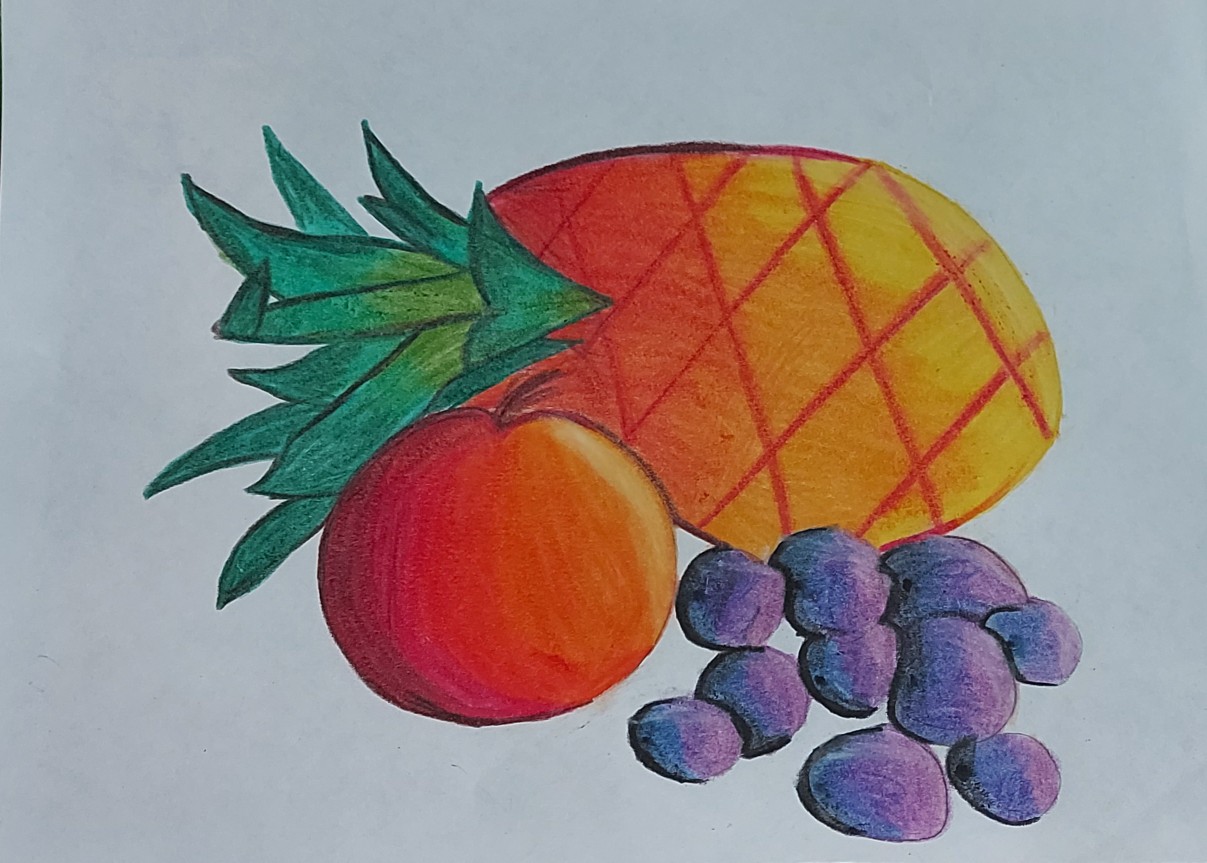This hand-drawn color image, created with crayons and colored pencils, features a lively arrangement of fruit against a light gray background. Dominating the composition is a pineapple lying on its side, with its green serrated leaves pointing to the left. The body of the pineapple transitions from a deep red at the top to a vibrant yellow at the bottom, and is covered with red crisscrossing lines. In front of the pineapple, positioned towards the left, is a round apple with hues that blend from pinkish-red on one side to yellow on the other, adorned with a small brown stem at the top. To the right of the apple, there is a cluster of purple grapes, each detailed with a small black dot at the top and encircled by a defining black outline. The artwork is set on a rectangular canvas, accentuating the vivid colors and intricate details of the fruit.